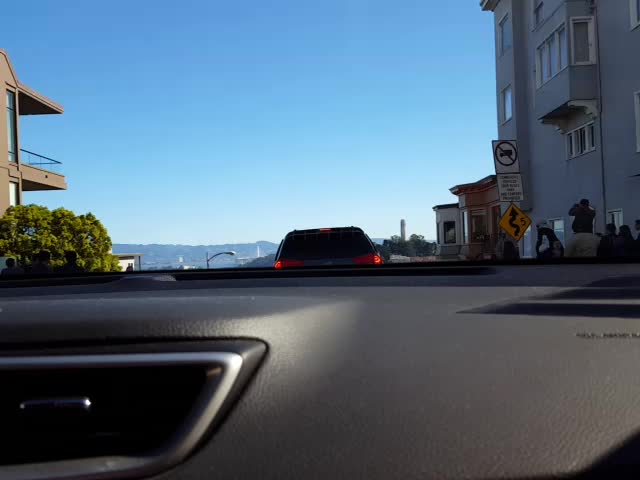This color photograph captures a cityscape as seen from inside a vehicle, looking out through the front windshield from what appears to be the top of a hill. The car's dashboard, visible at the bottom of the frame, features a silver-trimmed vent against a dark surface. Directly ahead, a car with its brake lights on dominates the foreground. To the left of the dashboard, a green air freshener tree hangs, while a brown building with a balcony can be seen. On the right, the scene reveals a larger blue building with numerous windows stretching upward. Below, a small group of people are walking past, next to a set of street signs – a prominent yellow one indicating a crooked road, and two white signs above it, one with a truck in a red circle. Further beyond, the scenery includes a small brown house, a white house, and a distant mountain range beneath a clear, blue sky. The sky is cloudless, enhancing the depth and clarity of the landscape.